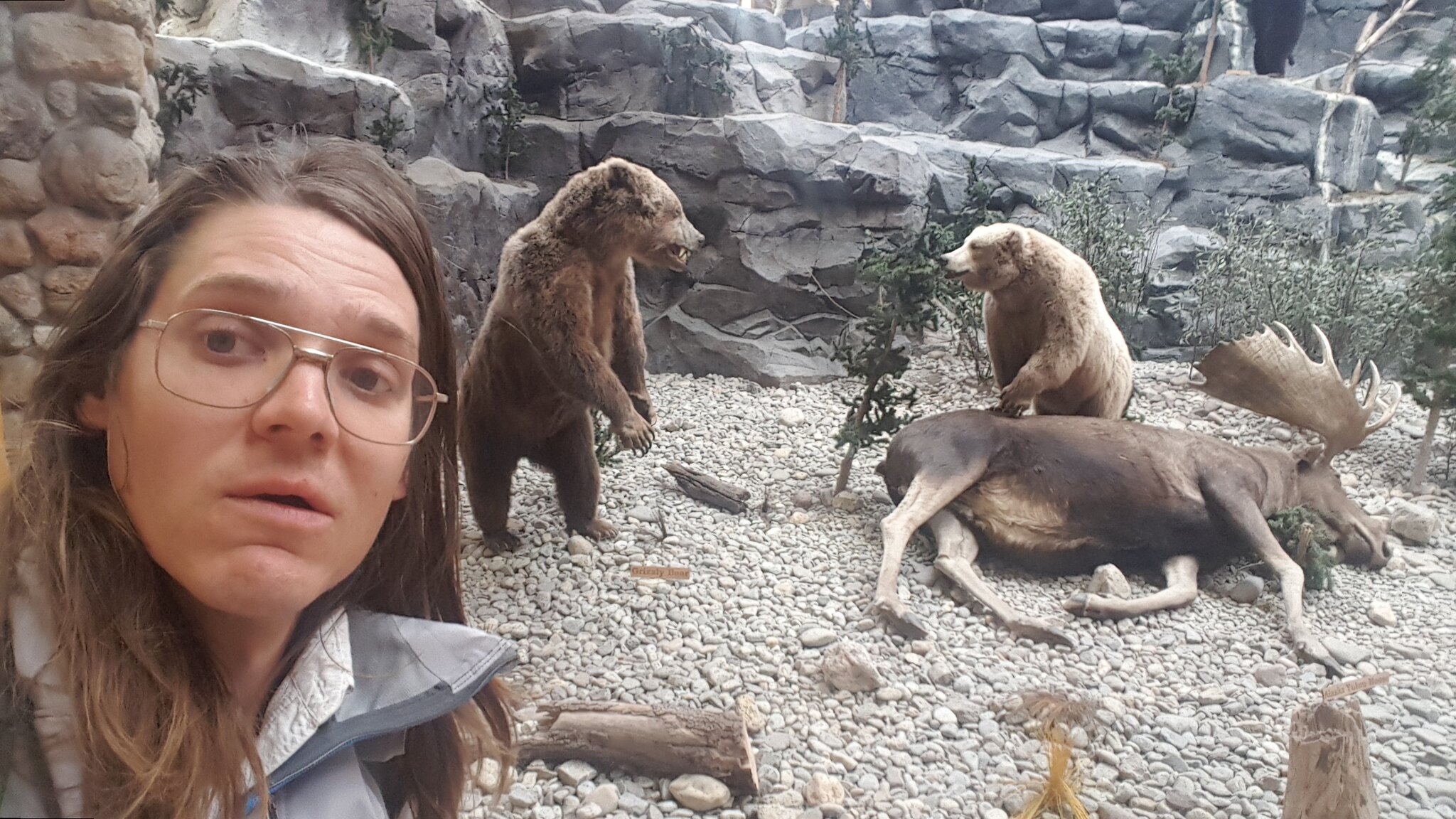In the foreground of the image, a person with long, dark hair and distinctive thin, gold-rimmed glasses gazes off to the left, not directly into the camera. They wear a light gray rain jacket with a wide collar that is open and lined with dark edging and white on the inside. This close-up captures them from the neck upwards, their expression a mix of curiosity and perplexity, as though they might be taking a selfie. 

Behind this individual, the scene unfolds against a backdrop resembling an artificial zoo exhibit of jagged, gray rocky outcrops, scattered with gravel stones and scrub, punctuated by a couple of fallen logs. Central to the composition are two large, brown bears. The bear on the left stands fully upright on its hind legs, facing slightly inward with its mouth partially open. The bear on the right, also on its hind legs but hunched over, faces its counterpart, adding a sense of interaction between the two animals.

On the ground before the right bear lies a moose, splayed on its left side with its majestic antlers and head raised, positioned slightly to the right of the frame. This setup, appearing almost like a museum exhibit with its surreal quality, suggests that the image has likely been manipulated or photoshopped, blending elements to create an unusual and striking outdoor scene.